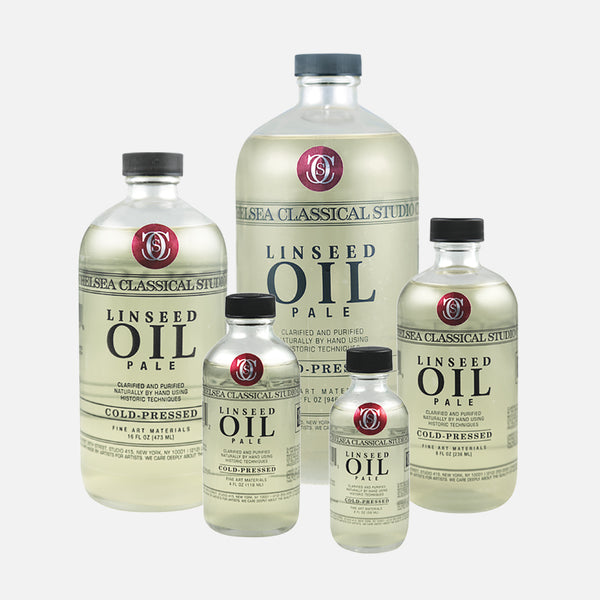In the center of the image with a light blue background are multiple transparent bottles of linseed oil, arranged by size. In this vertical rectangular composition, the largest bottle is placed in the middle, framed by slightly smaller bottles on its left and right. Further in the foreground, to the left and right of the central arrangement, are the smallest bottles. Each bottle seamlessly transitions from a broad cylindrical base to a narrower neck, capped with a round black top. 

Every bottle features a clear label bearing the text in what appears to be Times New Roman font. At the top of the label is a red oval logo, within which two overlapping white "C"s form a design encircling an "S". The primary label text reads "LC Classical Studio" across two horizontal lines at the top and "Linseed Oil Pale" prominently below. In smaller text beneath that, it states "Clarified and purified naturally by hand using historic techniques." Proceeding further down, additional text in Times New Roman font notes "Cold Press," bookended by more horizontal lines. Lastly, there are details about fluid ounces in block text near the bottom, although some of this text is obscured.

The arrangement and the consistent presentation of identical labels suggest a product advertisement, emphasizing the craftsmanship and quality of Chelsea Classical Studio's linseed oil.